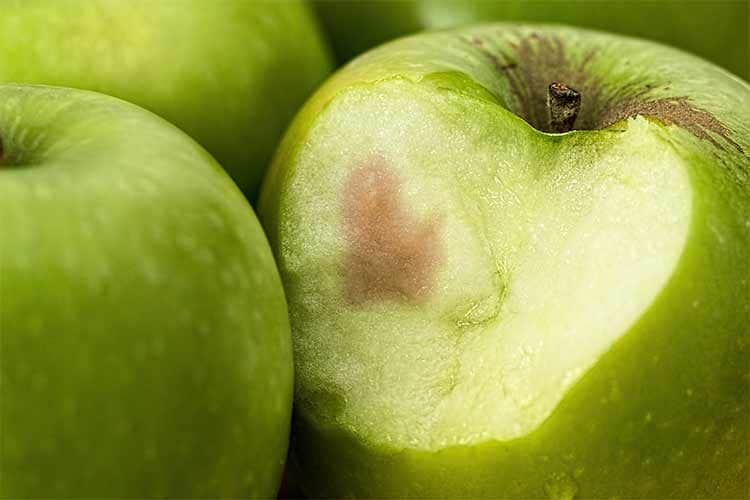The image is a horizontal rectangular photograph of four green Granny Smith apples. The background is dark, casting a shadowy effect over the entire scene. The featured apple dominates the right side of the picture, with a large bite taken out of its left side, revealing a brownish bruise surrounded by lighter off-white flesh. This apple also shows some brown discoloration around the stem, further indicating its age. The other three apples in the background are partially visible; they are bright green with lighter speckled spots and appear unblemished. The entire composition emphasizes the stark contrast between the freshness of the whole apples and the aged, bitten one.